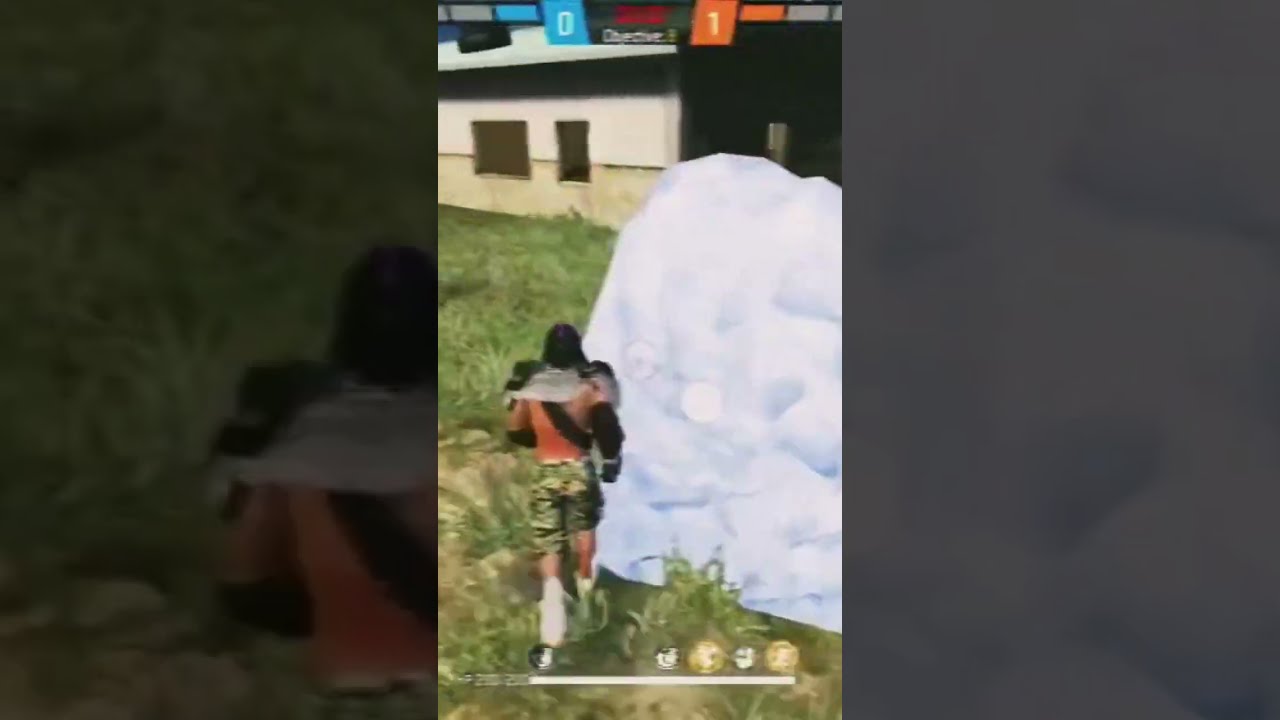In this image, which appears to be from a video game, we see a character wearing jungle camouflage pants, a red top, gray shoulder pads, and white shoes. The character has a black hood and is equipped with armor covering his shoulders and a strapped-on right arm, as well as knee guards. He is positioned in a grassy area, moving towards a two-toned building with a light white-gray top half and a light yellow bottom half. The building features two windows, a small square one and a larger horizontal rectangular one. To the right of the character, there is a large mound of white matter with blue shadows, possibly resembling snow or ice. 

At the top of the image, a scoreboard is visible showing a blue "0" on the left and an orange "1" on the right, with a timer or objective indicator in between. The image is flanked by grayed-out, zoomed-in sections of the main view, enhancing the focus on the central scene. This scene likely represents a competitive aspect of the game, with various status indicators and objectives displayed. The overall composition suggests an outdoor setting in the game, with clear visual elements that depict a tactical or action-oriented environment.